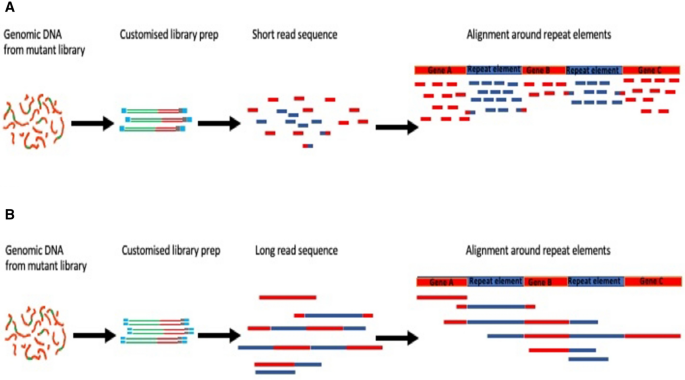The image depicts a detailed scientific diagram illustrating the sequencing process of genomic DNA from a mutant library, comparing short read and long read sequencing methods. At the top of section A, the flow begins with "genomic DNA from mutant library," represented by red and green squiggly lines. An arrow points toward the "customized library prep," where sequences are depicted as horizontal lines with blue ends and varying lengths of red and green. Another black arrow transitions into "short read sequence," illustrated by small, fragmented red and blue rectangles. These fragments are then aligned around repeat elements, with annotations indicating specific, though unreadable, textual details among the red and blue rectangles.

In section B, the diagram mirrors the steps in section A, starting again with "genomic DNA from mutant library" followed by "customized library prep." Unlike section A, the flow then proceeds to "long read sequence," shown as elongated red and blue rectangles. The final alignment around repeat elements here exhibits longer, continuous red and blue strips, contrasting with the shorter, fragmented alignment in section A. This comparison highlights the differences between short and long read sequencing in analyzing the genomic DNA from the mutant library. The overall diagram emphasizes the customization, sequencing, and alignment processes in DNA analysis, underscoring the contrasting outputs of short and long read sequencing technologies.